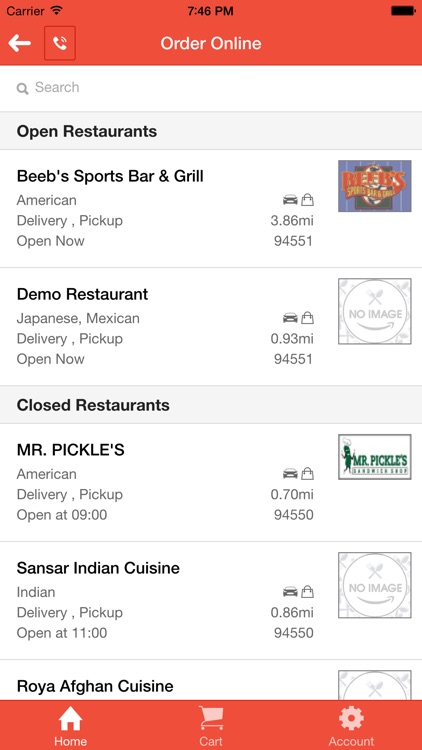The image depicts a mobile app interface designed for ordering food online, likely from a food delivery service. The screen is divided into two sections: one for open restaurants and another for closed restaurants. 

In the open restaurants section, four listings are fully visible, showcasing the following establishments: **Beeb's Sports Bar and Grill**, **Demo Restaurant**, **Mr. Pickles**, and **Sansar Indian Cuisine**. Information provided for each restaurant includes the type of cuisine they offer, their distance from the user, and the opening time for the following day. A partially visible fifth listing at the bottom of this section is **Royal Afghan Cuisine**, but no details about its open status are available.

The closed restaurants section marks restaurants as closed and not accepting orders. At the very top of the screen, there is a search bar that allows users to find additional information or search for specific restaurants.